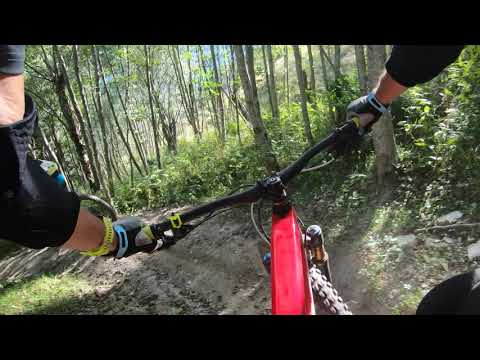This rectangular, full-color photograph, framed with thin black borders on the top and bottom, captures an outdoor scene during a sunny day. The image, taken from the perspective of a GoPro strapped to the photographer’s chest, shows a red mountain bike with black handlebars as it rides down a rugged dirt trail. The trail curves sharply to the left, winding through a dense forest of green trees and shrubs. The rider, whose arms are central to the composition, wears a short-sleeved black t-shirt, black elbow pads, and black gloves with blue wrists. A yellow bracelet adorns the rider's left wrist. Sunlight illuminates parts of the rider’s arms and the surrounding trees, clearly indicating daylight. The image vividly conveys the experience of biking through nature on a well-defined but challenging trail.